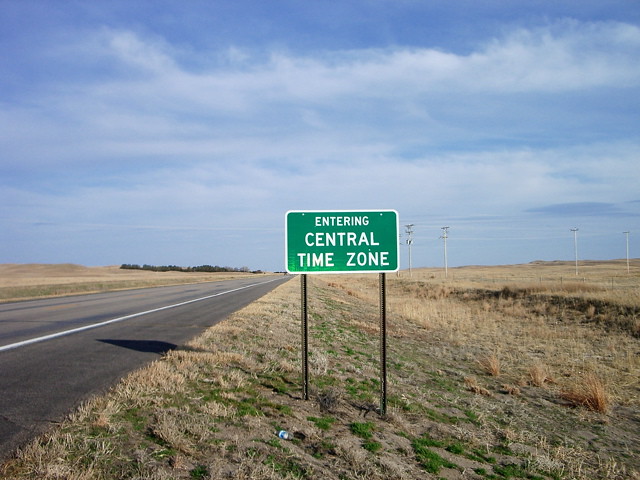In this image, a lonely two-lane road stretches out into a seemingly endless expanse of flat grasslands, fading into the horizon. The road is bordered by a low shoulder that slopes gently into the plain, which is covered with swathes of brownish grasses. Overhead, the sky is a serene blue, streaked with long, wispy clouds. On the far left side of the road, in the extreme distance, a faint tree line can be seen, while power lines run parallel to the road on the right side, drawing the eye towards the vanishing point. Prominently displayed in the foreground is a green informational sign, mounted about four feet off the ground, measuring roughly three feet in length and one and a half to two feet in width. The sign clearly indicates that you are "Entering Central Time Zone," though it doesn't specify from which direction you are coming. This evocative scene captures the essence of remote travel across vast, open lands.